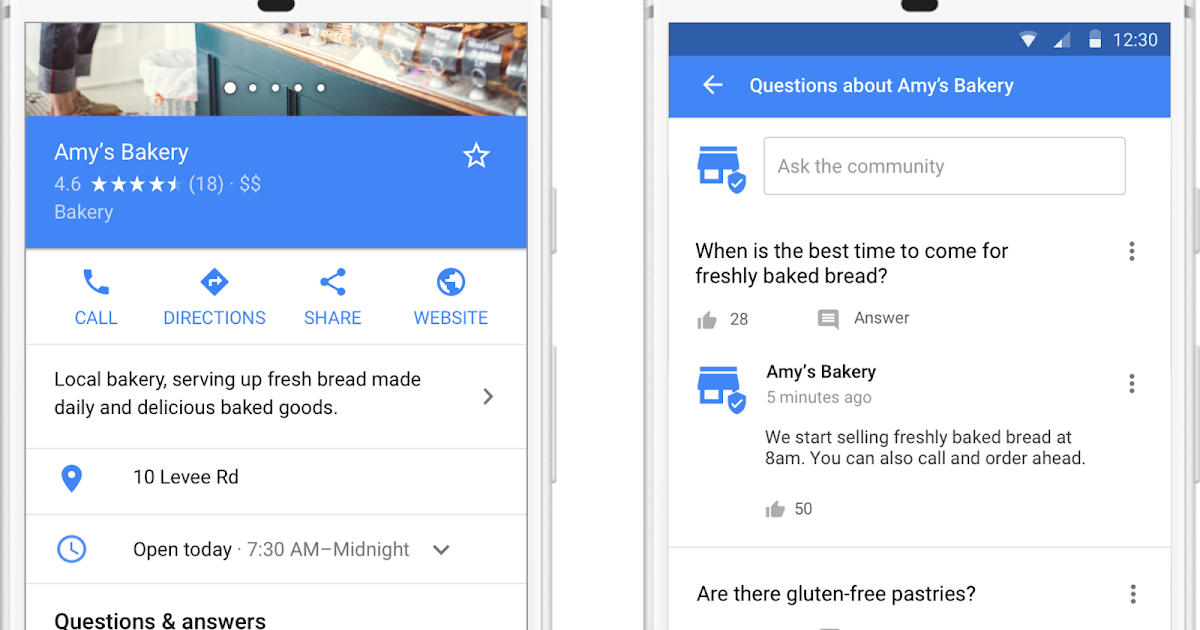The image depicts a cell phone displaying two screenshots related to Amy's Bakery. The phone has a sleek, light silver or white edge, giving it a modern aesthetic. 

The left screenshot shows a detailed profile of Amy's Bakery. At the top is an image of a countertop with a person standing on the left side. Below the image, a blue bar indicates "Amy's Bakery," rated 4.6 stars, classified as a bakery. The bakery’s description reads: "Local bakery serving up fresh bread made daily and delicious baked goods." The address provided is "10 Levee Road." Additionally, a clock symbol indicates the bakery's hours: "Open today, 7:30 a.m. to midnight." Below this information, there is a section titled "Questions and Answers."

The right screenshot features a Q&A section for Amy's Bakery. A blue bar at the top reads "Questions about Amy's Bakery." Below is a box prompting users to "Ask the community." The first question, in black text, asks, "When is the best time to come for freshly baked bread?" A response from Amy's Bakery, marked with a blue restaurant symbol and check mark, reads: "We start selling freshly baked bread at 8 a.m. You can also call and order ahead." This response has received 50 likes, indicated by a thumbs-up icon. At the bottom of the screen, another user question asks, "Are there gluten-free pastries?"

The detailed depiction provides a comprehensive look at the bakery's profile and interactive customer engagement.